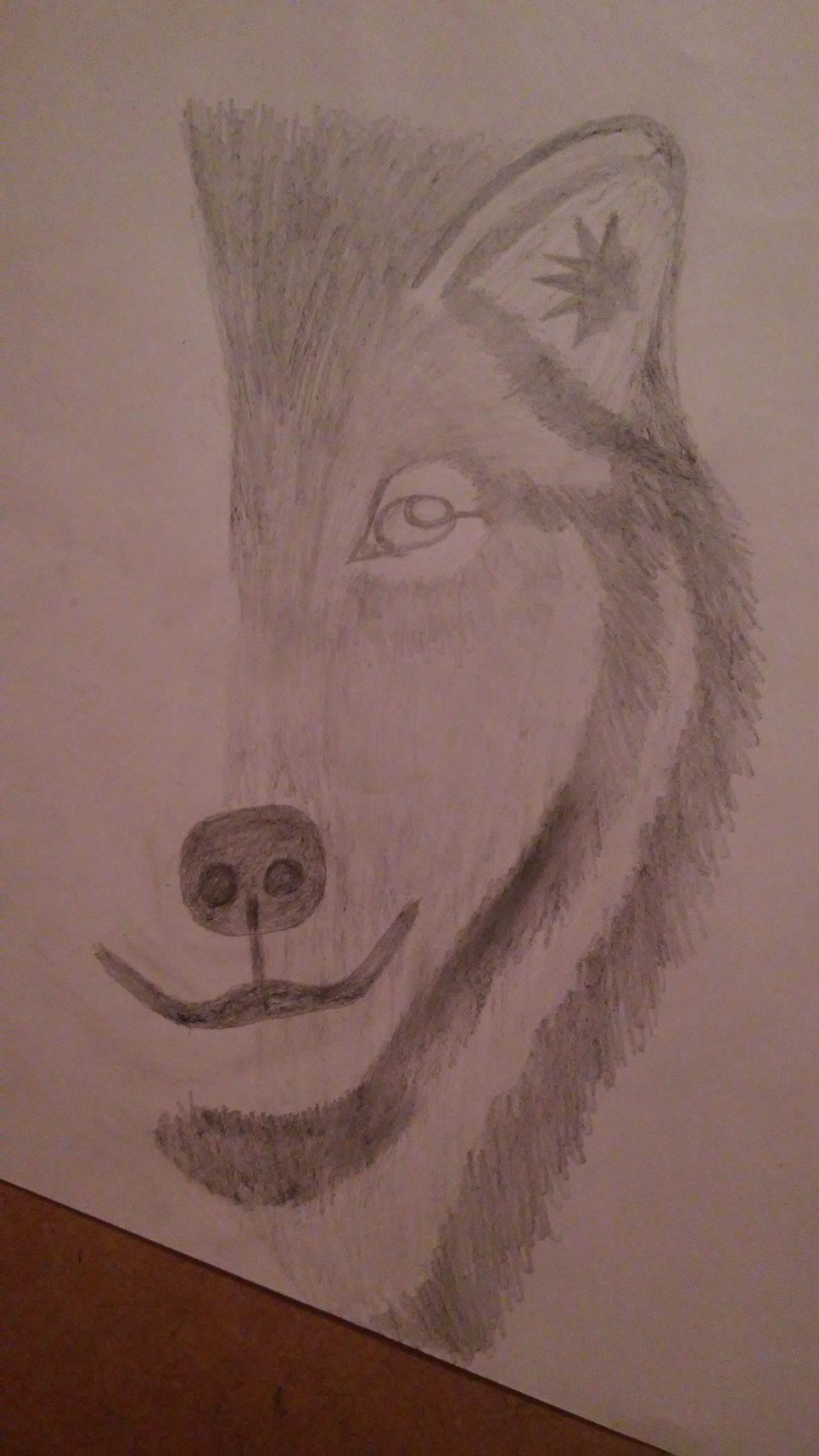This detailed pencil sketch in black and white captures most of a wolf's head, prominently showcasing its intricate fur texture. The fur is meticulously shaded, with lighter gray tones around the lower face transitioning into darker hues above the ear. Inside the ear, a notable detail is a small symbol resembling a star or sun. The wolf’s mouth is closed but subtly curves upward, giving the impression of a gentle smile. The left portion of the drawing remains incomplete, suggesting that the artist is still in the process of finalizing the artwork.